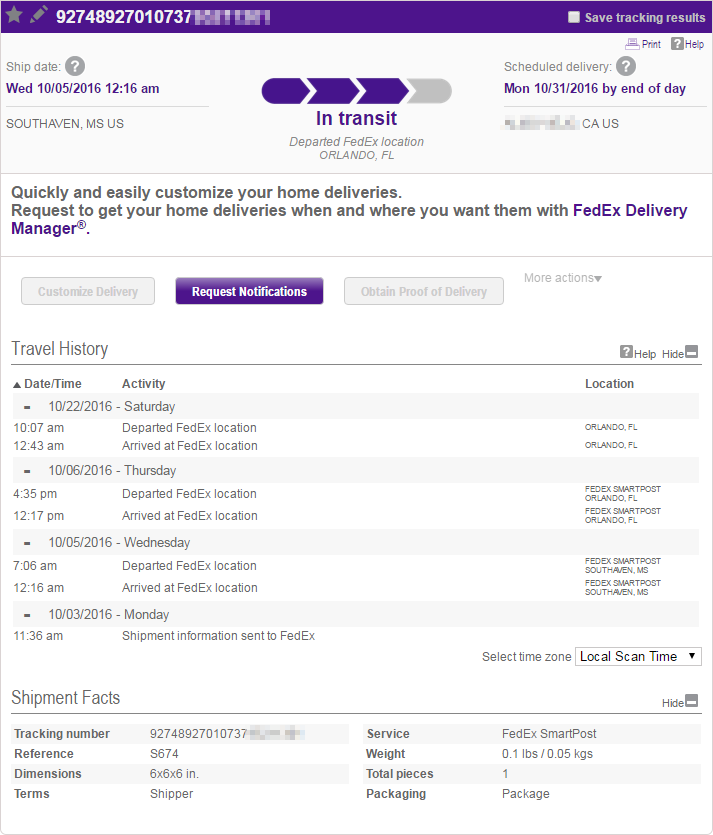**Descriptive Caption:**

At the top of the image, there is a purple-bordered section featuring three icons: a star, a pencil, and the number "92748927010737." To the right of these icons, the text reads "Save Tracking Results." Below this, a label titled "Ship Date" appears next to a gray circle with a question mark in its center. Beneath this, it indicates "Wednesday 10/05/2016 at 12:16 AM." Further to the right, the status "In Transit" is displayed, specifying that the package "Departed FedEx location in Orlando, Florida." The scheduled delivery is set for "Monday 10/31/2016 by the end of the day." An informative message follows, encouraging users to "quickly and easily customize your home deliveries" and "request to get your home deliveries when and where you want them with FedEx Delivery Manager."

Below this message, there are three buttons: a gray one labeled "Customize Delivery," a purple one that says "Request Notifications," and another gray one stating "Obtain Proof of Delivery."